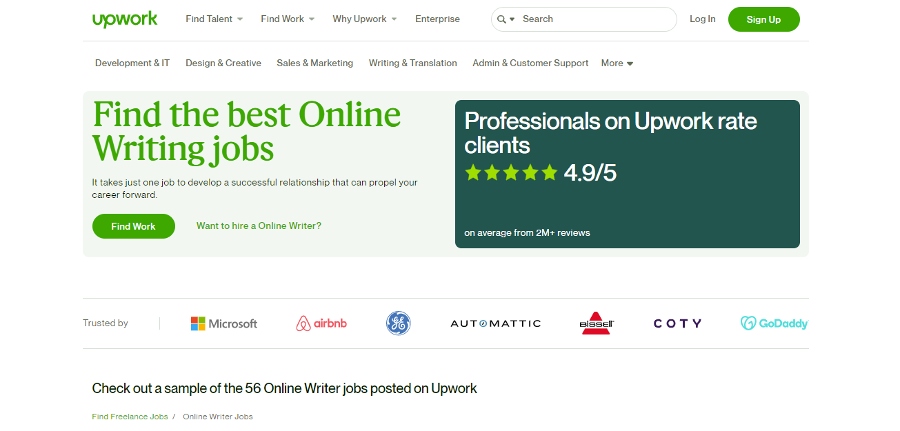This is a screenshot from the Upwork website. At the top, the word "Upwork" is displayed in green small caps. Beside it, there are links labeled "Find Talent," "Find Work," "Why Upwork?" and "Enterprise." A search bar is prominently featured along with "Log In" and "Sign Up" options. The "Sign Up" button is white text on a green rectangular background with rounded edges. 

Directly below, there are clickable categories for different types of work: "Development & IT," "Design & Creative," "Sales & Marketing," "Writing & Translation," "Admin & Customer Support," and more.

A highlighted section reads, "Find the best online writing jobs" in green text set against a very light green background, followed by a motivational line: "It takes just one job to develop a successful relationship that can propel your career forward." Another button reiterates, "Find Work."

Adjacent to this, a dark green text box with white lettering states, "Professionals on Upwork rate clients 4.9 out of 5 stars on average, from over 2 million reviews." This is accentuated with five green stars.

Below this text box, the companies "Microsoft," "Airbnb," "Automatic," "Bissell," "Coty," and "GoDaddy" are listed under "Trusted by," suggesting their endorsement. Finally, the page mentions, "Check out a sample of 56 online writer jobs posted on Upwork," inviting users to explore job opportunities.